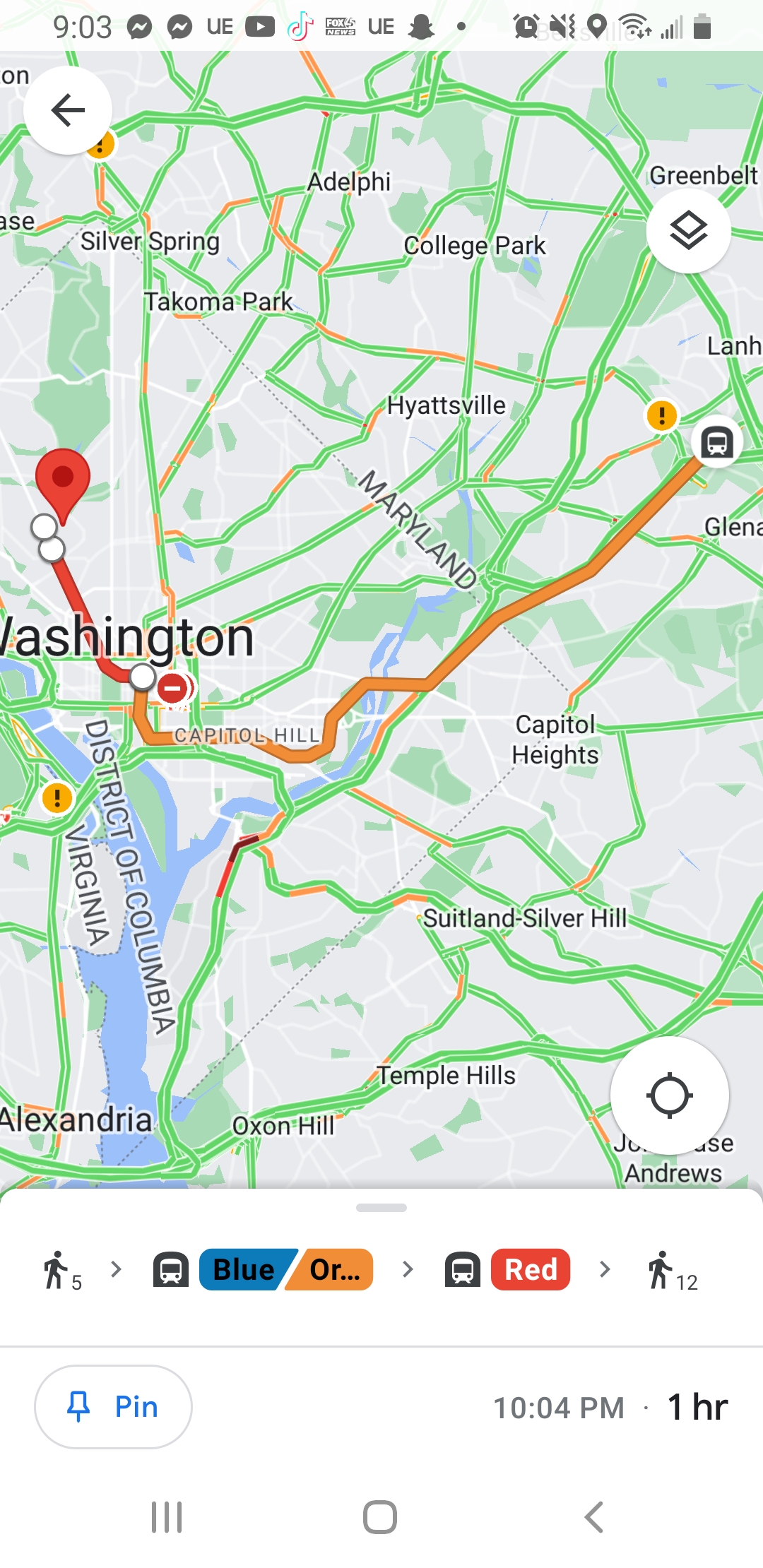This image is a screenshot of an iPhone displaying directions for using public transportation in Washington, DC. It is in portrait orientation with approximately 95% occupied by a detailed map. The map prominently features Washington, DC in the center, with the first three quarters of the 'W' truncating on the left edge. Located at the top right of the map is Maryland, while the District of Columbia and Virginia are positioned at the bottom of the map. Various green roadways, depicted in bright green, crisscross the area, and an orange line represents a specific bus route. This route begins on the center-right of the map, moves left across Capitol Hill, and continues to the left before concluding at an upside-down red teardrop icon, indicating the destination.

The top of the screen displays the current time, 9:03 a.m., along with several app icons in gray. At the bottom are the written directions beneath the map: the user is instructed to walk for 5 minutes, take a bus route identified by blue/orange labels to the red bus, and then walk for an additional 12 minutes. The total travel time is indicated to be one hour, with the expected arrival time being 10:04 p.m.